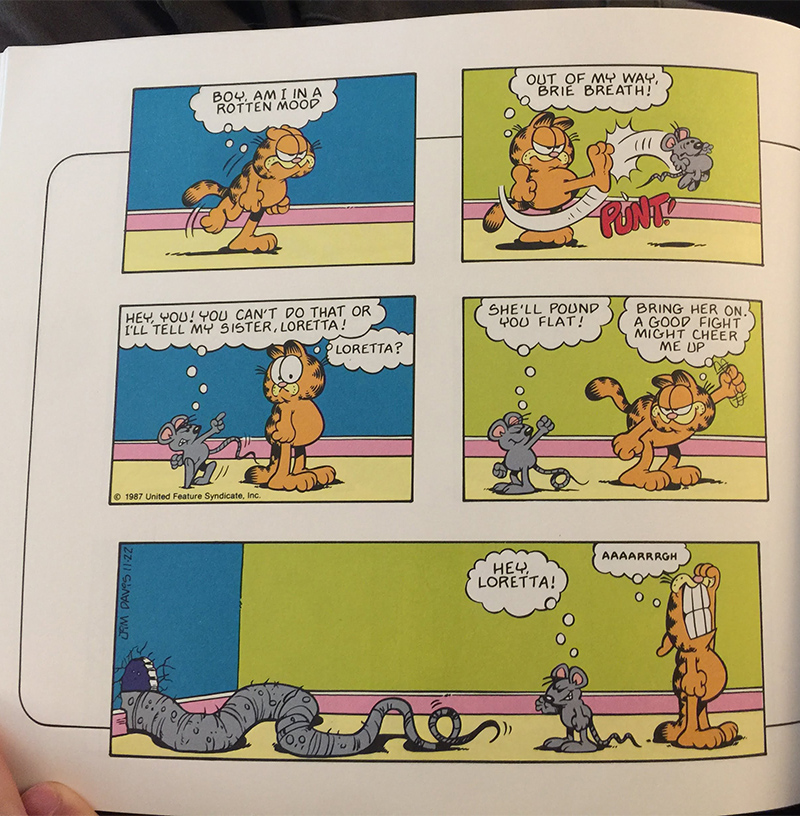The image is an open book featuring a 1987 Garfield comic strip by Jim Davis. The strip comprises five panels against a gradient background starting with a yellow floor, transitioning through various colors including pink, blue, and green.

The first panel sets Garfield in a room with a blue wall and a pink stripe, declaring, "Boy, I'm in a rotten mood" in a white text bubble. The second panel shows Garfield kicking a gray mouse with the word "PUNT" in red beneath his foot, while he says, "Out of my way, breathe breath." The third panel shows the mouse retaliating, "Hey you, you can't do that or I'll tell my sister Loretta," to which Garfield, thinking, "Loretta," looks perplexed. In the fourth panel, the mouse warns, "She'll pound you flat," and Garfield, undeterred, replies, "Bring her on, a good fight might cheer me up."

The final panel spans the bottom of the strip and reveals a large, snaking tail emerging from a mouse hole, implying Loretta’s enormous size. The mouse calls, "Hey Loretta," while Garfield reacts with an exasperated "ARGH," conveying his sudden apprehension. The image includes a visible hand turning the page, adding a touch of realism to the comic strip scene.